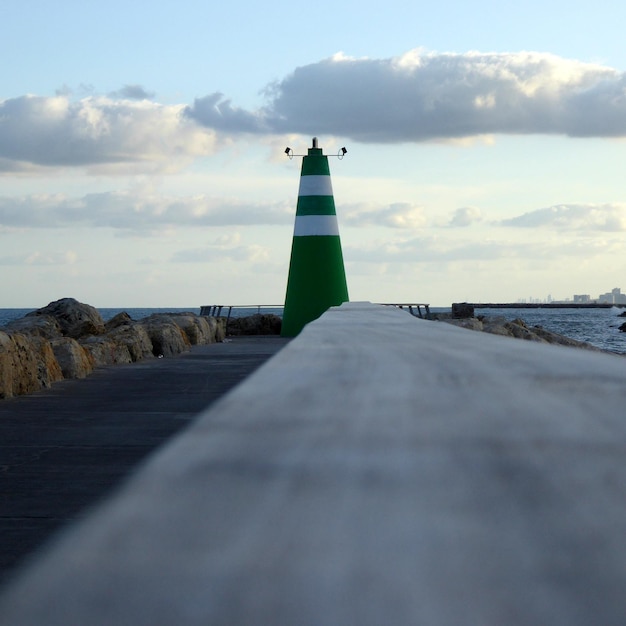In this image, a small, green, conical-shaped lighthouse with two white stripes near its top stands prominently at the end of a concrete pier or walkway extending into a calm ocean. The lighthouse's unique design, reminiscent of the top of a green Crayola crayon, suggests its function despite its unconventional appearance. Large boulders flank the pier, offering protection and leading up to the base of the lighthouse. The scene is viewed from a blurred foreground, possibly from behind a railing, emphasizing the lighthouse at center stage. The horizon showcases tranquil blue waters with minimal waves and a distant cityscape peeking out from the right-hand corner. The sky above is a soft blue with scattered white clouds, suggesting a late afternoon setting.